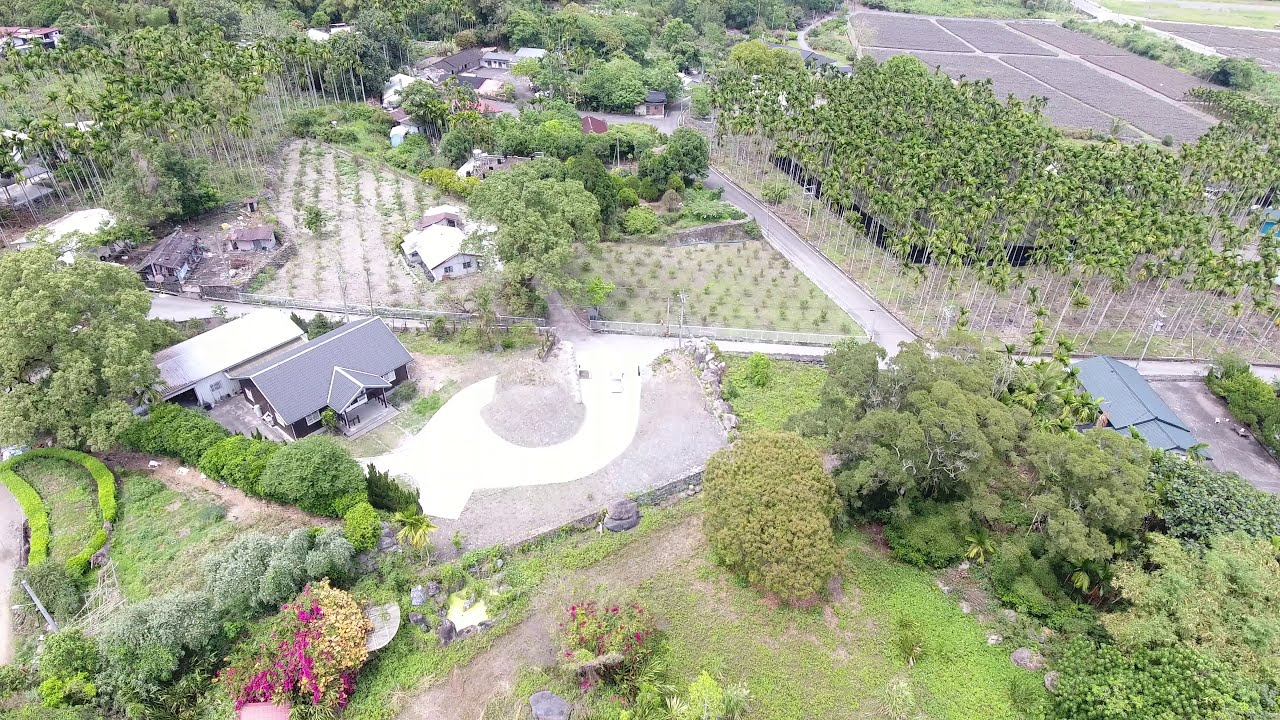This overhead shot captures a rural tropical neighborhood, divided into various plots of land. On the left side of the image stands a dark brown house with a gray, framed roof, surrounded by lush gardens, flowering bushes, and other greenery. Adjacent to this house is a white building with a flat roof. In the center, a horizontally-running dirt or single-lane road bisects the area.

Around the middle of the photograph, a distinctive circular driveway, strikingly white against the tan-colored dirt, features prominently. On the other side of the road lie several smaller rural houses and their corresponding plots, interspersed with dense trees, including numerous tall, slender, white-trunked palm trees with bushy green tops. In the background, especially on the top right, several plots are organized into small farm parcels. The area teems with green foliage, reinforcing its tropical ambiance.